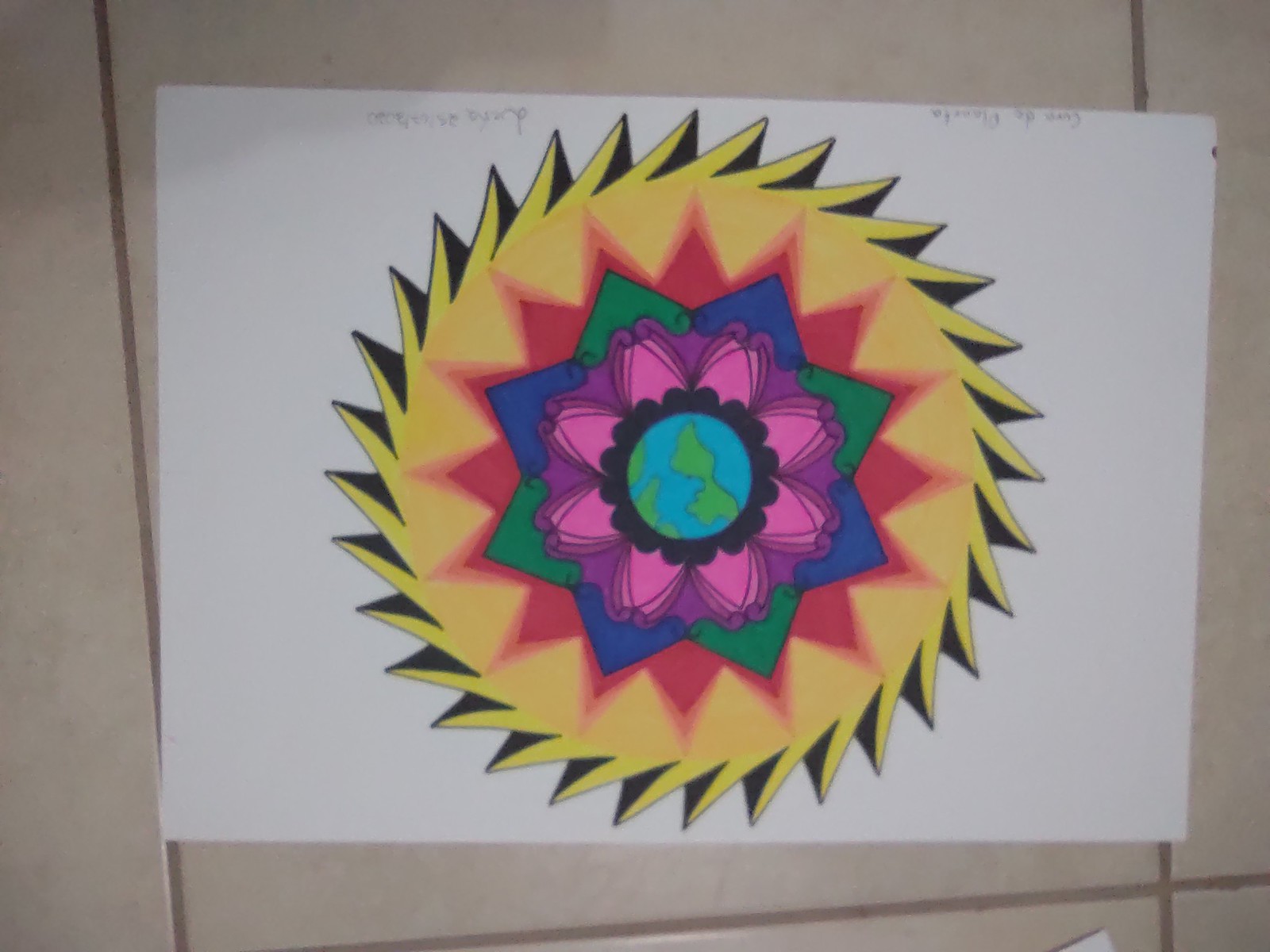The image depicts a detailed, circular mandala design on a white piece of paper, which is placed on a gray tiled floor. The mandala resembles the sun with its yellow outer edges featuring little sunray-like extensions. Encircling the design is a black border that gives it a gear or wheel-like appearance. 

Within this border, the mandala progresses inward through various vibrant colors and shapes: starting with light orange, followed by overlapping green and blue squares, and then a series of repeating red triangles forming a flower-like shape. Further inward, there is a concentric pattern made up of alternating purple and pink elements. At the very core of the mandala lies a small, detailed depiction of the planet Earth, with blue for the water and green indicating the landmasses. 

Additionally, some fine handwriting in pencil on the paper includes signatures and perhaps the name of the piece, although they are difficult to decipher due to their small size and the quality of the photo. The overall presentation of the drawing suggests it might be a school project, possibly created by an older elementary or middle school student. The photograph of the drawing appears to be taken from a top-down perspective, emphasizing the intricate and colorful details of the mandala.